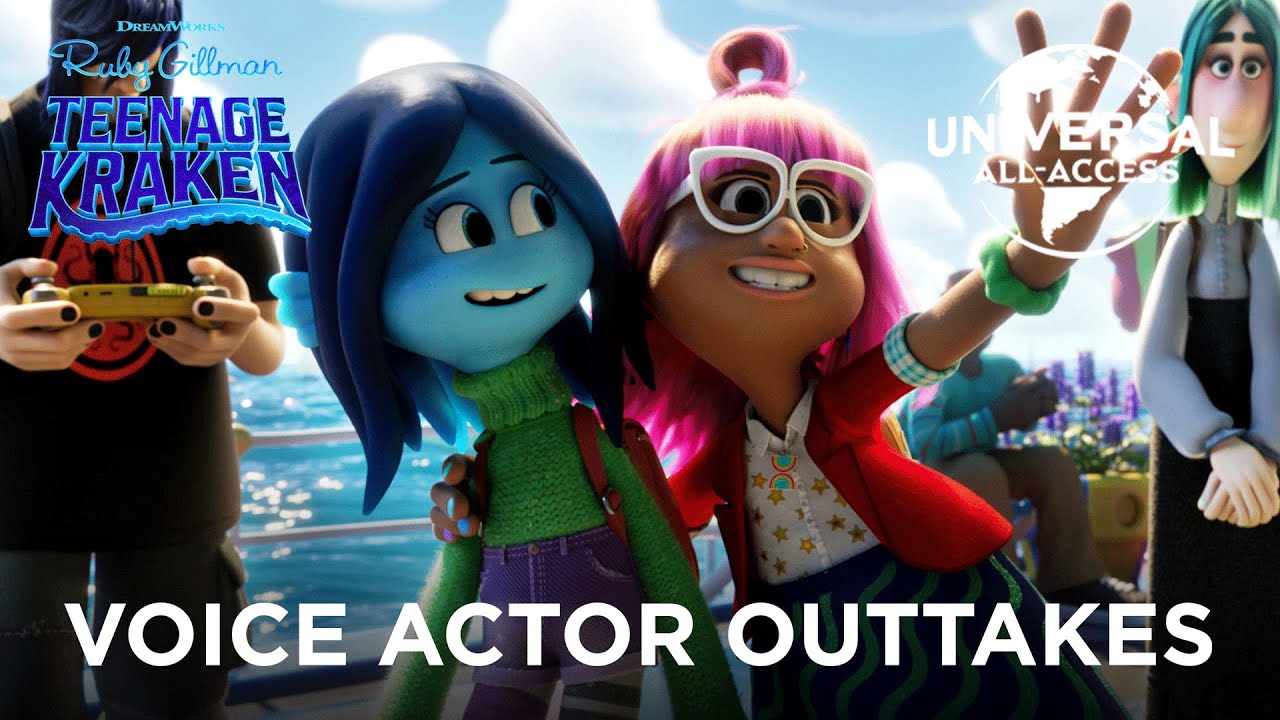The image is a horizontal rectangular scene from the computer-animated movie "DreamWorks Ruby Gillman, Teenage Kraken." It features four cartoon characters standing on the deck of a ship, indicated by the visible railing, with a vast blue sky and large clouds in the background. In the foreground, two young women, one with pink hair and her arms spread wide as if waving, and the other with blue skin and blue hair, are prominently placed. Accompanying them are two other characters: a little boy standing on the left side and another woman on the right side, who has green hair. Along the bottom of the image, large white text reads "Voice Actor Outtakes," while the upper left corner displays "Teenage Kraken" in bold blue letters outlined in aqua. On the upper right corner, there is a white circle with "Universal All Access" emblazoned within it. The overall scene gives the impression of a joyful moment captured on a cruise ship with clear blue waters in the distance.